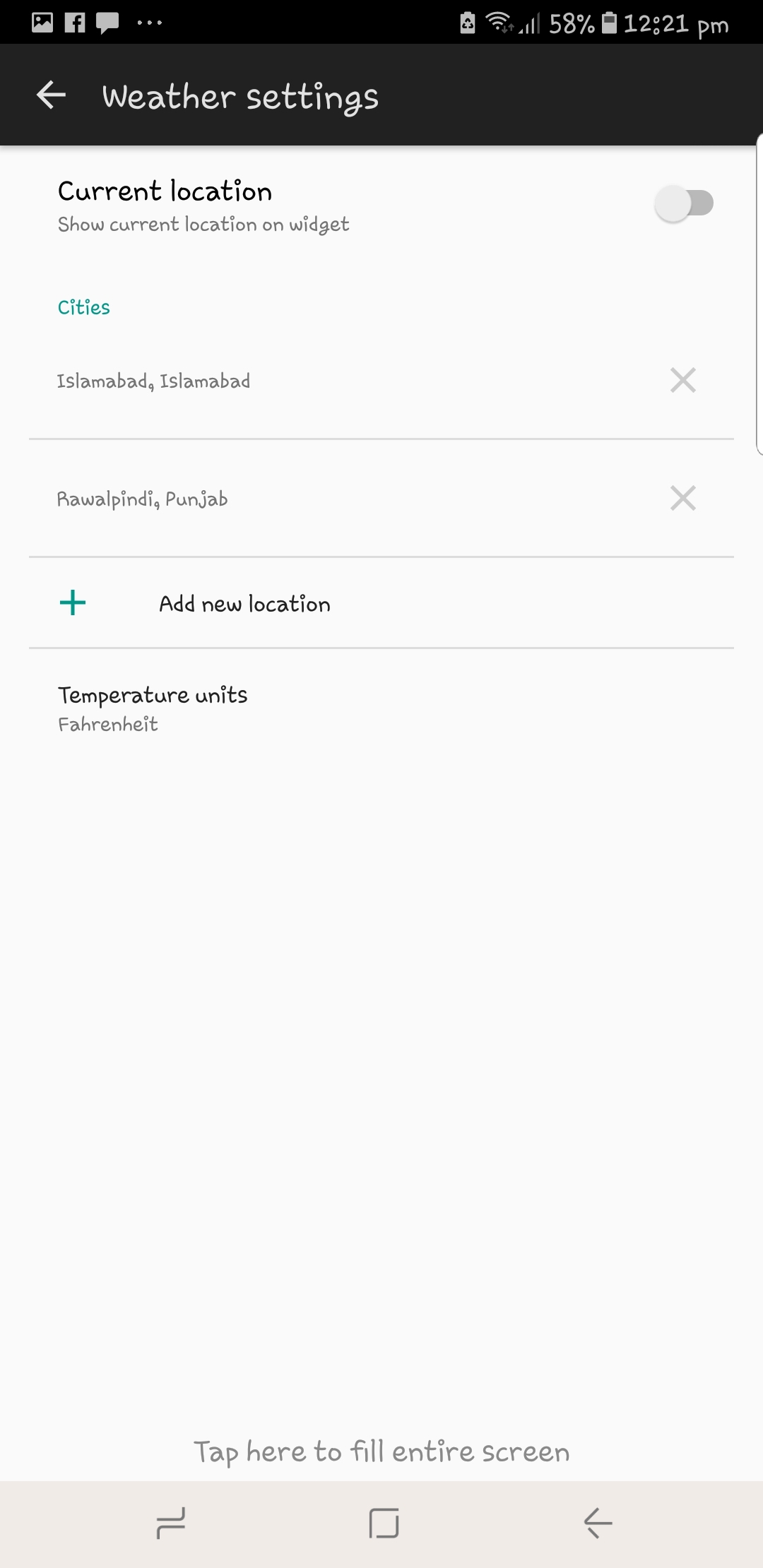This image is a screenshot of the weather settings screen from a mobile phone. At the very top, the status bar features a black background with various icons. On the right side, there is a battery icon showing 58% and the time marked at 12:21 PM. The left side of the status bar displays icons for Facebook, portrait orientation, and messages. 

Directly below the status bar is a black header titled "Weather Settings." Beneath this header, the main content is presented on a white background that resembles a drop-down window. The first option is "Current Location," with a toggle switch next to "Show current location on widget" that is turned off.

The next section lists cities, highlighted in blue. The first city listed is "Islamabad," accompanied by an 'X' on the far right for deletion. This is followed by another city located in Punjab, also featuring an 'X' for removal at the far right. After the listed cities, there is a section with a blue plus sign labeled "Add new location."

Towards the bottom of the screen, there is a setting for "Temperature Unit" set to Fahrenheit. A relatively large gap separates the sections, and at the very bottom center of the screenshot is a prompt saying, "Tap here to fill entire screen."